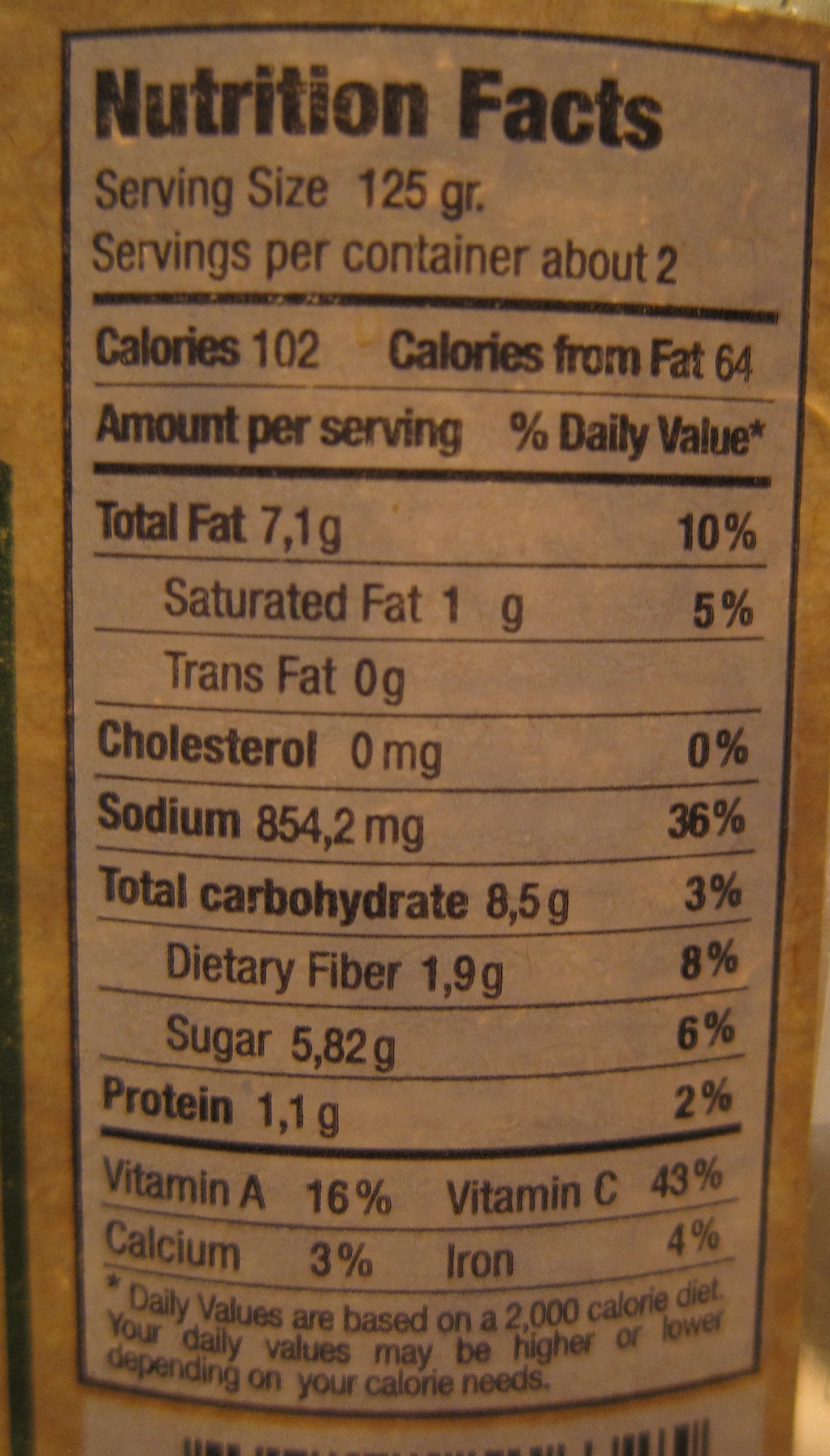The image depicts an old-fashioned brown label, resembling brown packing paper, showing the nutritional content of an unspecified product. At the top of the label, "Nutritional Facts" is written in dark, bold type. The serving size is listed as 125 grams, with approximately 2 servings per container.

Beneath a dark line, the label details the caloric content: 102 calories per serving, with 64 calories from fat. The "Amount Per Serving" percentage and daily value information are also in bold type. Another bold line separates this section from the following specific nutrient details:

- Total Fat: 7.1 grams (10% of daily value)
- Saturated Fat: 1 gram (5%)
- Trans Fat: 0 grams
- Cholesterol: 0 milligrams (0%)
- Sodium: 8.54 milligrams (0.2%)
- Total Carbohydrate: 8.5 grams (3%)
- Dietary Fiber: 1.9 grams (8%)
- Sugars: 5.82 grams (6%)
- Protein: 1.1 grams (2%)

Another bold line follows, separating the vitamin and mineral content listed below:

- Vitamin A: 16%
- Vitamin C: 43%
- Calcium: 3%
- Iron: 4%

At the bottom of the label, a note clarifies that the daily values are based on a 2,000-calorie diet and may vary based on individual calorie needs.